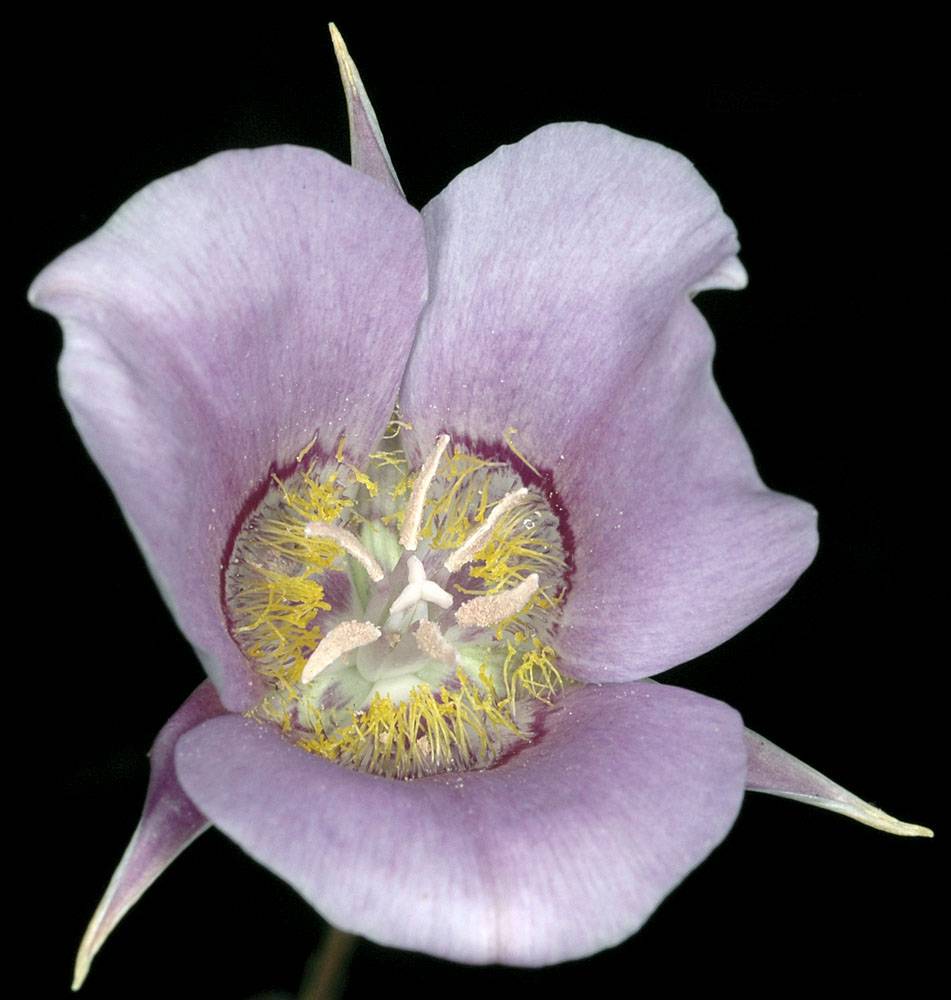This is a highly detailed close-up of a striking purple and white flower set against a pitch-black background. At the center of the flower, there is a white spot featuring a complex design with streaks and fibrous plant parts, likely designed to hold pollen. The center is encircled by a deeper, darker purple, adding depth and contrast to the overall appearance. The flower has three main petals that start with a medium purple hue near the center, gradually transitioning to very light purple or white towards the edges. Additionally, three pointed, propeller-like leaves extend behind these petals, lending further complexity to the structure. Surrounding the central white spot are six delicate hairs, white and light peach in color, while thin, long, yellow hairs are attached to the petals. The flower's overall symmetry and the stark black background make for a visually stunning image, with the black providing excellent contrast and emphasis on the intricate details and vibrant colors of the flower.